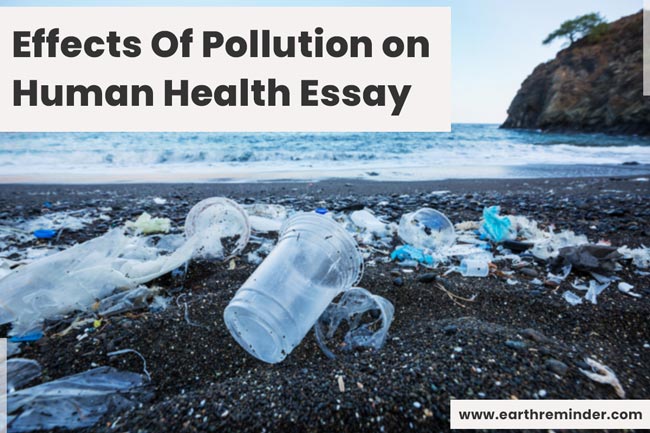The image is a horizontal landscape photograph depicting a polluted shoreline. The top third of the image features a white background with two lines of black text that read, "Effects of Pollution on Human Health Essay." In the bottom right corner, the website "www.earthreminder.com" is prominently displayed. The foreground of the photo reveals a beach littered with various types of plastic debris, including small microplastics, larger plastic containers, bottle caps, and bags. The beach itself is composed mainly of black rocks and pebbles, with minimal sand. In the upper right corner, there's a hill topped with a solitary tree. The background showcases a gradient light blue sky, suggesting a clear, sunny day. The overall image serves as a vivid illustration of environmental pollution.